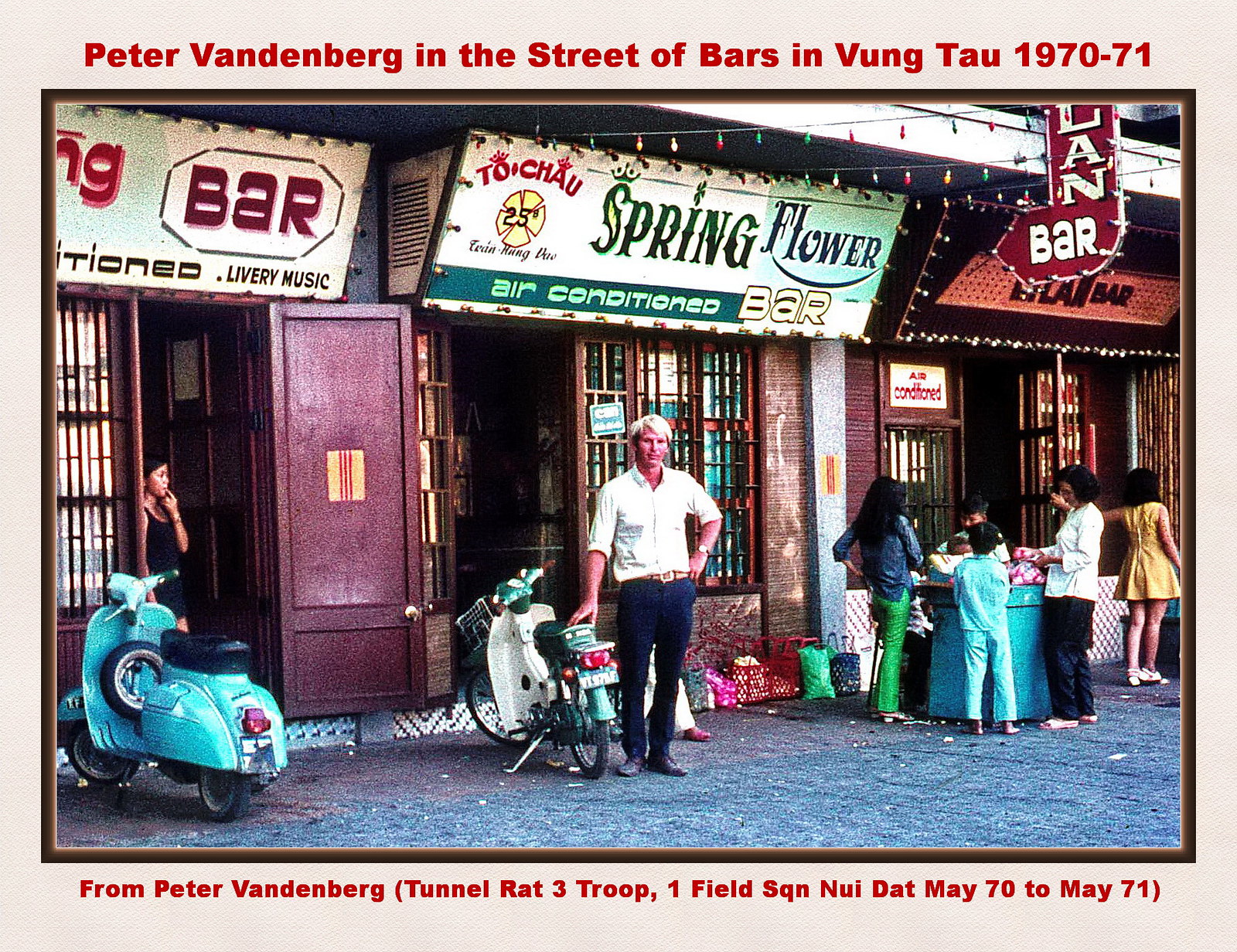This vintage framed photograph, inscribed in red lettering at the top with "Peter Vandenberg in the Street of Bars in Vung Tau, 1970 to 1971," captures a moment from the early 1970s. The image features a tall, blonde man identified as Peter Vandenberg, dressed in a white button-up shirt with rolled-up sleeves, blue jeans, and a belt. He poses confidently with one hand on his waist and the other resting on the seat of a light blue scooter, gazing directly at the camera.

The scene is set in front of the Springflower Air-Conditioned Bar, distinguishable by its green and white sign. Flanking this establishment on either side are additional bars, creating a bustling and vibrant street atmosphere. To the left of Peter stands a young Vietnamese woman in the bar’s doorway, while to the right, a group of local people, including women and children, gather around a table, adding to the lively ambiance.

The storefronts, with their clustered and busy appearance, feature brown wooden facades and bar windows, giving a glimpse into the social life of the area. Additional scooters, including a greenish-blue one on the far left, dot the foreground of this evocative snapshot of Vung Tau's nightlife during the Vietnam War era. At the bottom of the photograph, the inscription reads, "From Peter Vandenberg, Tunnel Rat 3 Troop, Field 1, May 1970-May 1971," providing further context to this historical image.